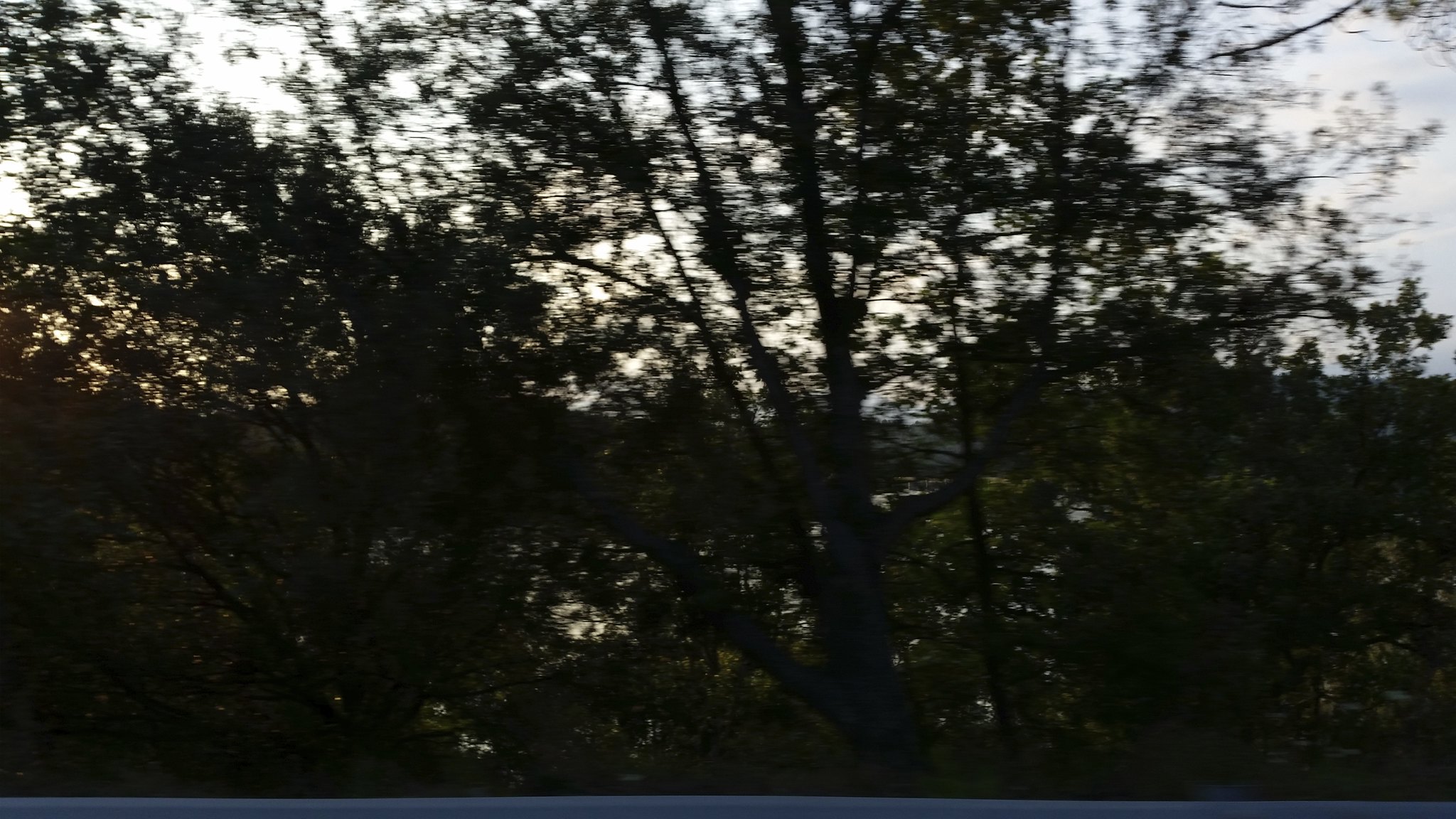The image is a very blurry, rectangular, and horizontal color snapshot of a woodland area, predominantly showcasing a dense collection of deciduous trees with green leaves and wide, gray-brown trunks. In the middle-right part of the background, there are hints of potential pine trees. The sky above is slightly overcast and blue, with dim light suggesting either dawn or dusk, contributing to the backlit, shadowy appearance of the tree line. Towards the left side, the sky takes on a faint orange hue, likely indicating a sunrise or sunset. Near the bottom third of the frame, there's an indistinct suggestion of water through the trees, though the blur makes it difficult to confirm. The overall scene is dark and somewhat obscured by the lack of focus, with no visible text or writing in the image.